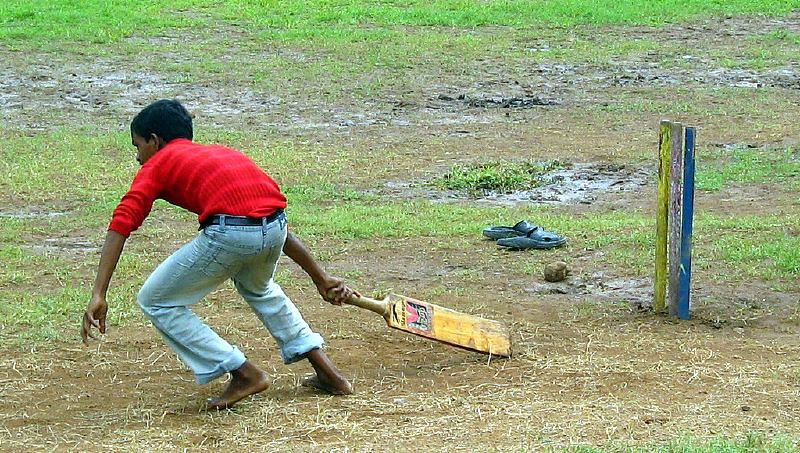The photograph captures an action shot of a cricket match on a muddy field dotted with wet puddles, suggesting recent rain. Dominating the left side of the horizontal rectangular image is a young boy with dark hair, dressed in blue jeans—rolled above the ankles and secured with a black belt—and a red ribbed long-sleeve shirt with the sleeves rolled up. He appears to have just hit the ball, as he is seen dropping the bat, which trails behind him, and starting to run. His blue sandals lie near the center of the image, beside a round leather cricket ball partially submerged in a puddle. Further to the right, three wooden posts stand closely together, each painted a different color—yellow, white, and blue—though the paint is worn and streaked with mud. The rest of the field in the background is a mix of green grass and muddy patches, completing the scene of a post-rainy day cricket match.